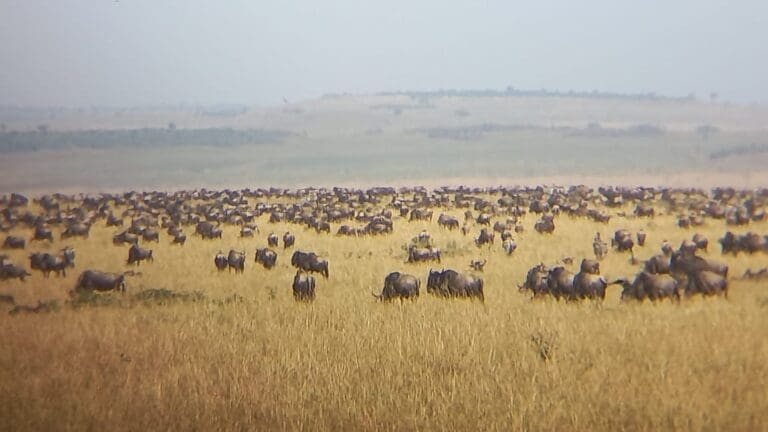The image depicts a vast prairie in the Great Plains under daylight, featuring thousands of buffaloes grazing. The foreground showcases a sprawling green grassland teeming with the brown and black forms of these majestic animals. In the background, higher prairies and distant hills are visible under a cloudy blue sky, which blurs slightly into the horizon. The scene is bathed in soft sunlight, accentuating the varied colors of greens, yellows, blues, grays, blacks, and whites across the expansive landscape. This setting embodies the serene and untamed wildlife characteristic of the American Great Plains.